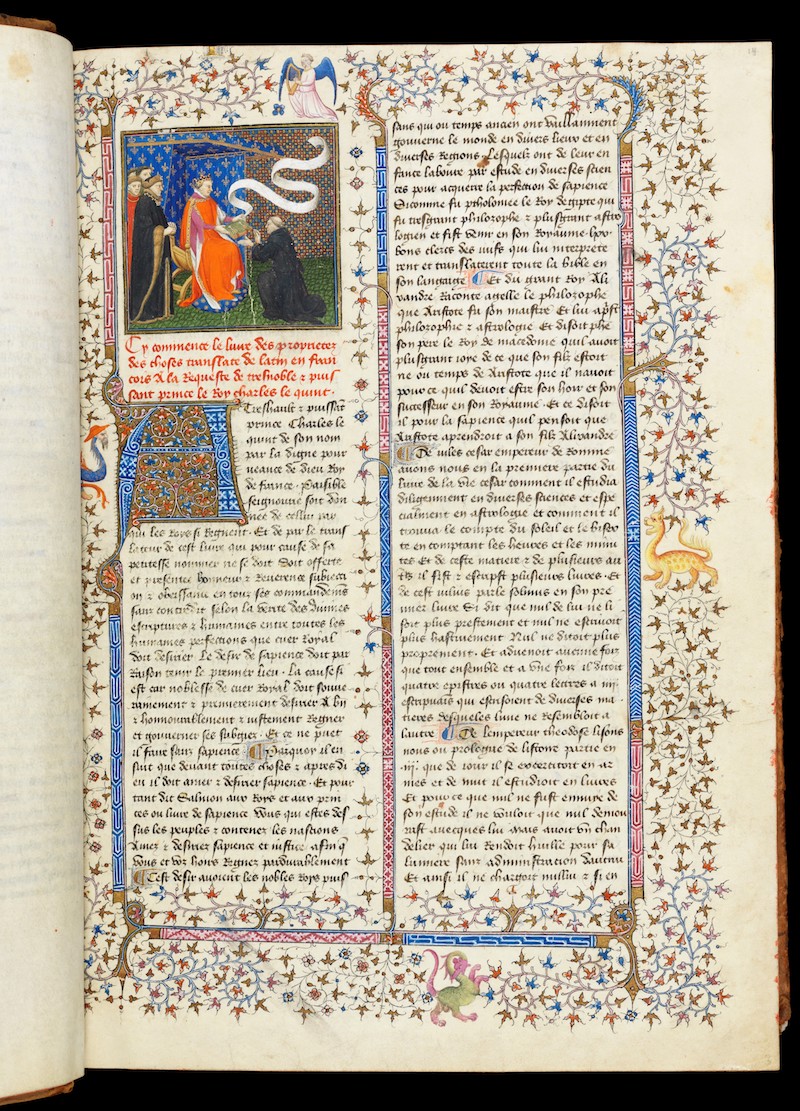This image showcases a single page from an ornate, medieval manuscript. The text appears to be written in an ancient or non-English language, potentially Welsh or Latin. The manuscript is richly decorated, featuring intricate designs of leaves and branches in vibrant blues, reds, pinks, and golds, framing the primary writing in the center. The writing itself is in calligraphy, beginning with a large, highly detailed initial 'A,' followed by tiny, meticulously rendered text in two columns. The ink transitions from red to black as it progresses. The margins of the page are adorned with elaborate, colorful illustrations, including dragons, an angel, and other fanciful creatures. In the upper left corner, there's an image of a scene depicting a figure in dark robes kneeling before another figure in red robes, possibly representing a friar and a king, with onlookers present in the background. The page shows signs of age, with a yellowed appearance, indicating its historical significance.